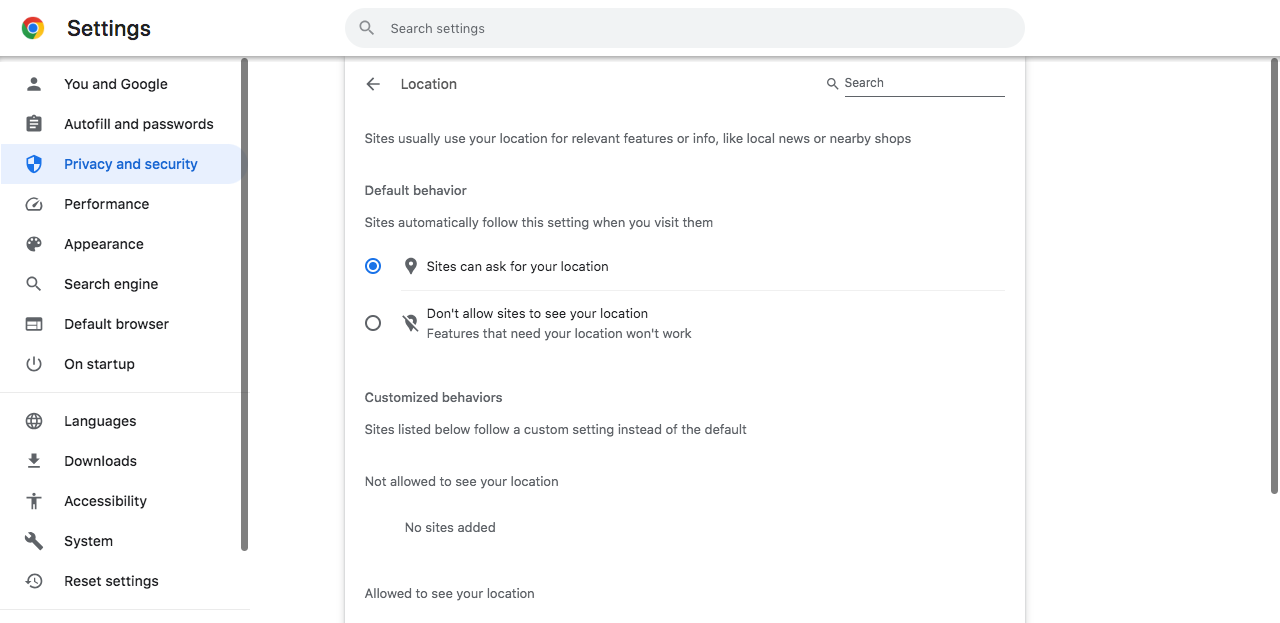This image displays the Google Chrome settings interface, easily identifiable by the familiar red, yellow, and green logo centrally placed within the browser window. The settings menu is open, revealing a vertical list of options that users can click to expand further information. Currently, the "Privacy and Security" section is selected, indicated by its highlighted blue background. This section is the third option from the top, preceded by "You and Google" and "Autofill and Passwords."

Within the "Privacy and Security" section, the screen showcases various privacy settings. At the top, there is an option for "Location," which prompts users to choose site-specific behavior for sharing location data. Below this, a descriptive note informs that websites typically use location data to provide relevant features or information.

Two primary settings are available under "Default behavior": one that allows sites to ask for the user's location and another that disallows any site from tracking location. The first option, permitting sites to request location access, is currently selected.

Further down, a section titled "Customized behaviors" lists individual site settings. This part includes headings like "Not allowed to see your location" (currently no sites are added under this heading) and "Allowed to see your location."

Beyond the "Privacy and Security" category, additional settings options are visible further down the menu, including "Performance," "Appearance," "Search Engine," "Default Browser," "On Startup," "Languages," "Downloads," "Accessibility," "System," and "Reset Settings."

This meticulously detailed presentation highlights the current focus on privacy settings within Google Chrome, offering users a glance at the browser's customizable security and privacy features.